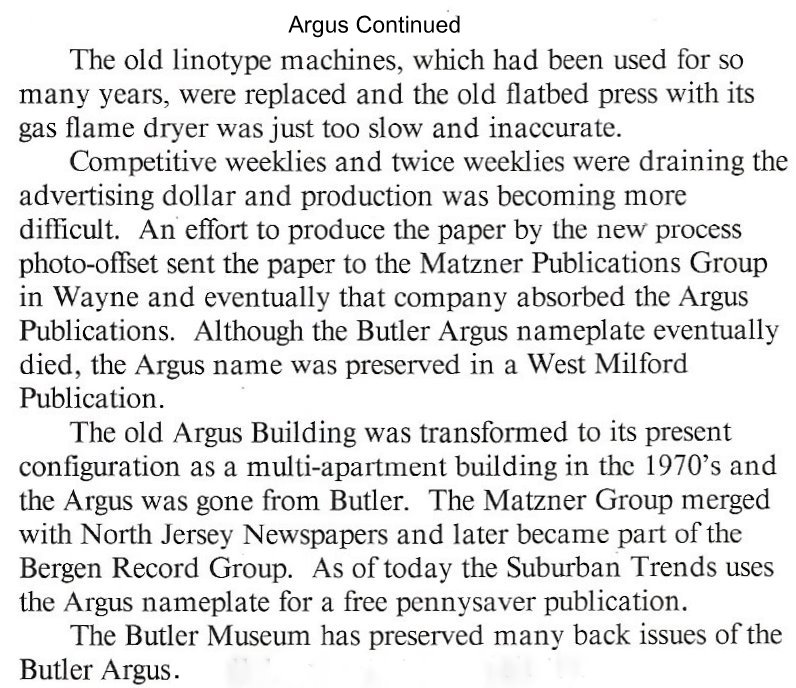This image is a scanned page from a book, featuring a white background with black text in sans-serif font. At the very top, the heading reads "Argus continued." Centered on the page, there's a heading that repeats "Argus continued," followed by a detailed paragraph. The paragraph describes how the old Linotype machines and the flatbed press with its gas flame dryer became outdated and inefficient. Due to increasing competitive pressures from weeklies and twice weeklies, there was a shift to using the new photo offset process. This transition led to the paper being incorporated into the Matzner Publications Group in Wayne, which eventually absorbed Argus Publications. Although the Butler Argus nameplate eventually became defunct, its name was preserved in a West Milford publication. The original Argus building was converted into a multi-apartment structure in the 1970s, marking the end of Argus in Butler. The Matzner group later merged with North Jersey Newspapers, becoming part of the Bergen Record Group. Currently, Suburban Trends uses the Argus name for a free penny saver publication. The final line mentions that the Butler Museum has preserved many back issues of the Butler Argus.